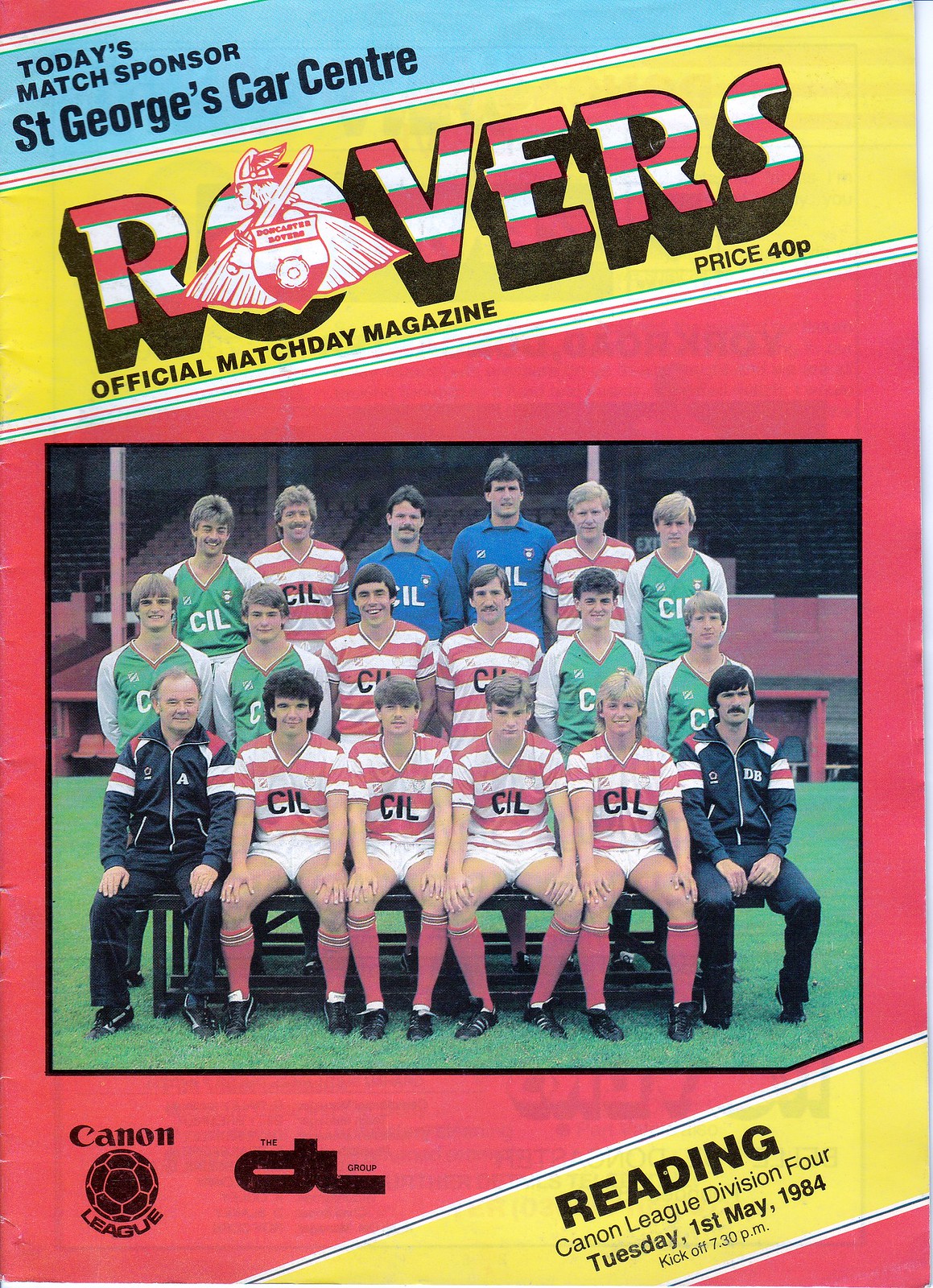The image is a scan of an official match day magazine cover for the Rovers, dated Tuesday, May 1st, 1984, for a Cannon League Division 4 game against Reading, with a kickoff time of 7:30 p.m. The magazine's title, "Rovers," is prominently displayed in bold red and white striped blocky letters with shadow effects, and the letter 'O' features a viking emblem depicting a side-view of a viking with a sword on his shoulder and a winged helmet. Above the title, a blue banner states the day's match sponsor, St. George's Car Center. Below the title, on a red background with a dark frame, there is a color photograph of the soccer team. The team photo shows players in red and white striped jerseys, some in green jerseys with v-neck collars, and two goalkeepers in blue jerseys. The coaches, positioned on the bottom left and right, are dressed in black track suits. The team is posed on a green field with stadium stands in the background. Additional details include the price of the magazine, 40p, located to the right of the title, and two sponsor logos on the bottom left corner. The overall style of the cover blends photographic realism with graphic design elements, suggesting a production approach from the 1980s.